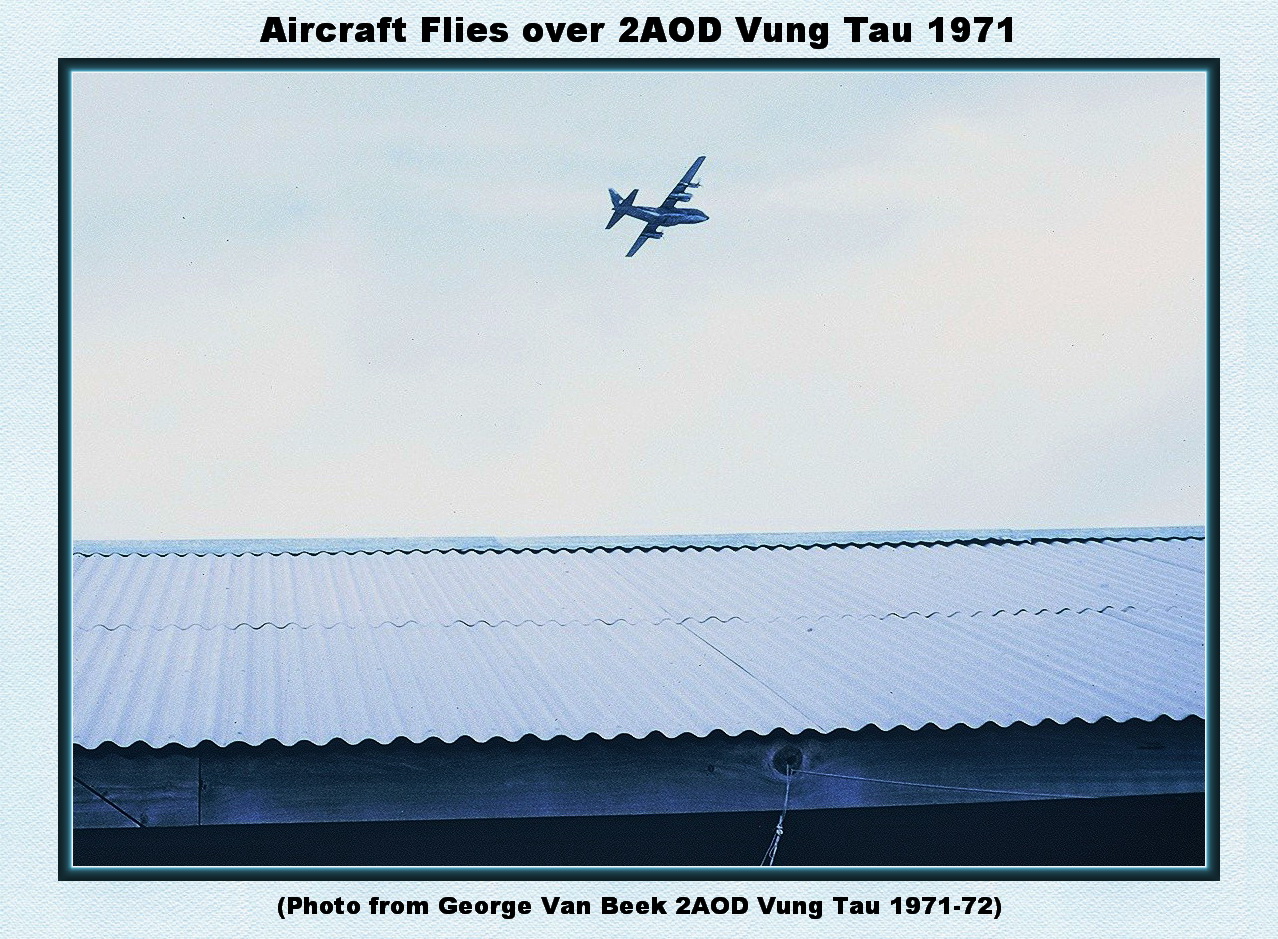This is a color photograph with a cool tone filter, predominantly in shades of pale blue, likely due to its age. The image captures a cloudy sky with an overcast appearance. At the center, a small airplane with four motors is seen turning left and slightly downward. The foreground features a corrugated sheet metal rooftop supported by wooden beams, with sections of the roof showing waves in the metal. The photograph has text in black on a light blue border; at the top, it reads "Aircraft Flies Over 2 A.O.D. Vung Tau 1971," and at the bottom, it says "Photo from George Van Beek, 2 A.O.D. Vung Tau, 1971-72."